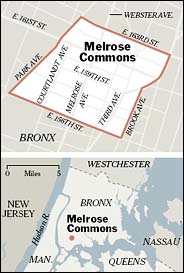This detailed graphic of Melrose Commons features a two-part vertical rectangle map. The upper half provides a close-up view of Melrose Commons, a roughly square area with a slight curvature on the right side and outlined in red. This close-up helps orient viewers by detailing the specific streets and borders within the Bronx. The lower half of the graphic displays a broader map showing where Melrose Commons is situated within the Bronx County. This part of the map includes neighboring regions for context: New Jersey on the left, the Hudson River, and New York State, with the Bronx prominently indicated in white. Surrounding areas such as Westchester County to the north, Queens to the south, and Nassau County to the southeast are also marked. This dual-level depiction effectively situates Melrose Commons within the larger geography of the region.